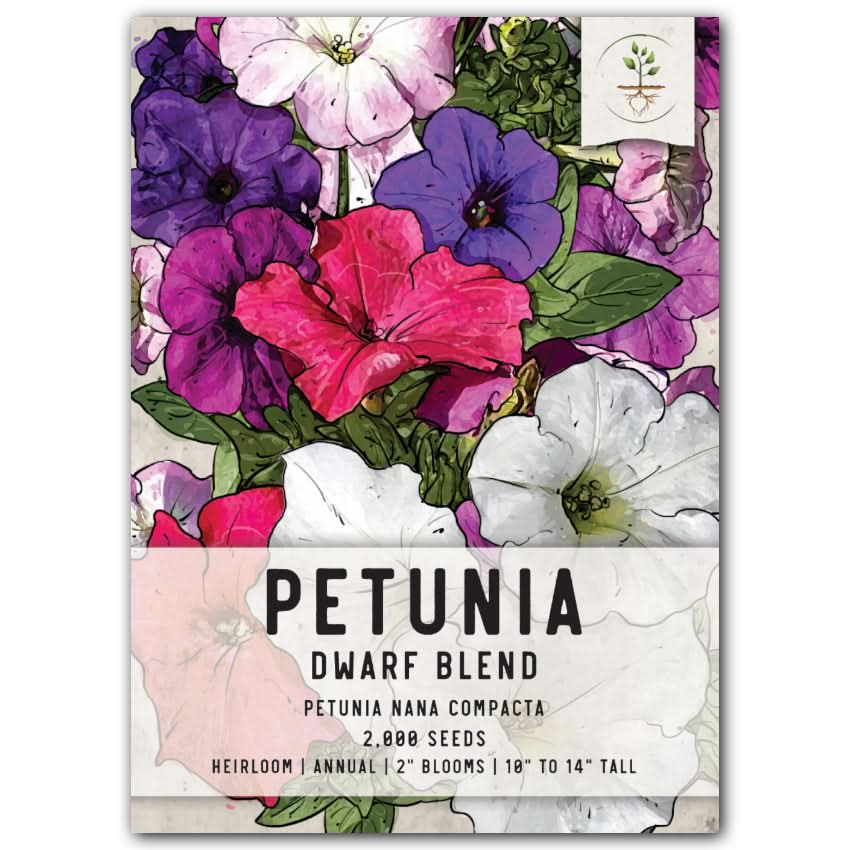This detailed colored drawing appears to be the front cover of a seed packet for "Petunia Dwarf Blend." The text at the bottom, arranged in five lines, reads: "Petunia Dwarf Blend, Petunia Nana Compacta, 2,000 Seeds, Heirloom, Annual, 2-inch Blooms, 10-inch to 14-inch Tall." The bottom half of the image features a bouquet of petunias with a variety of flower colors, including red, white, purple, and blue, surrounded by lush green leaves. In the top right corner, there is a tag displaying an illustration of a plant, with its roots visible beneath the soil and five leaves growing above.